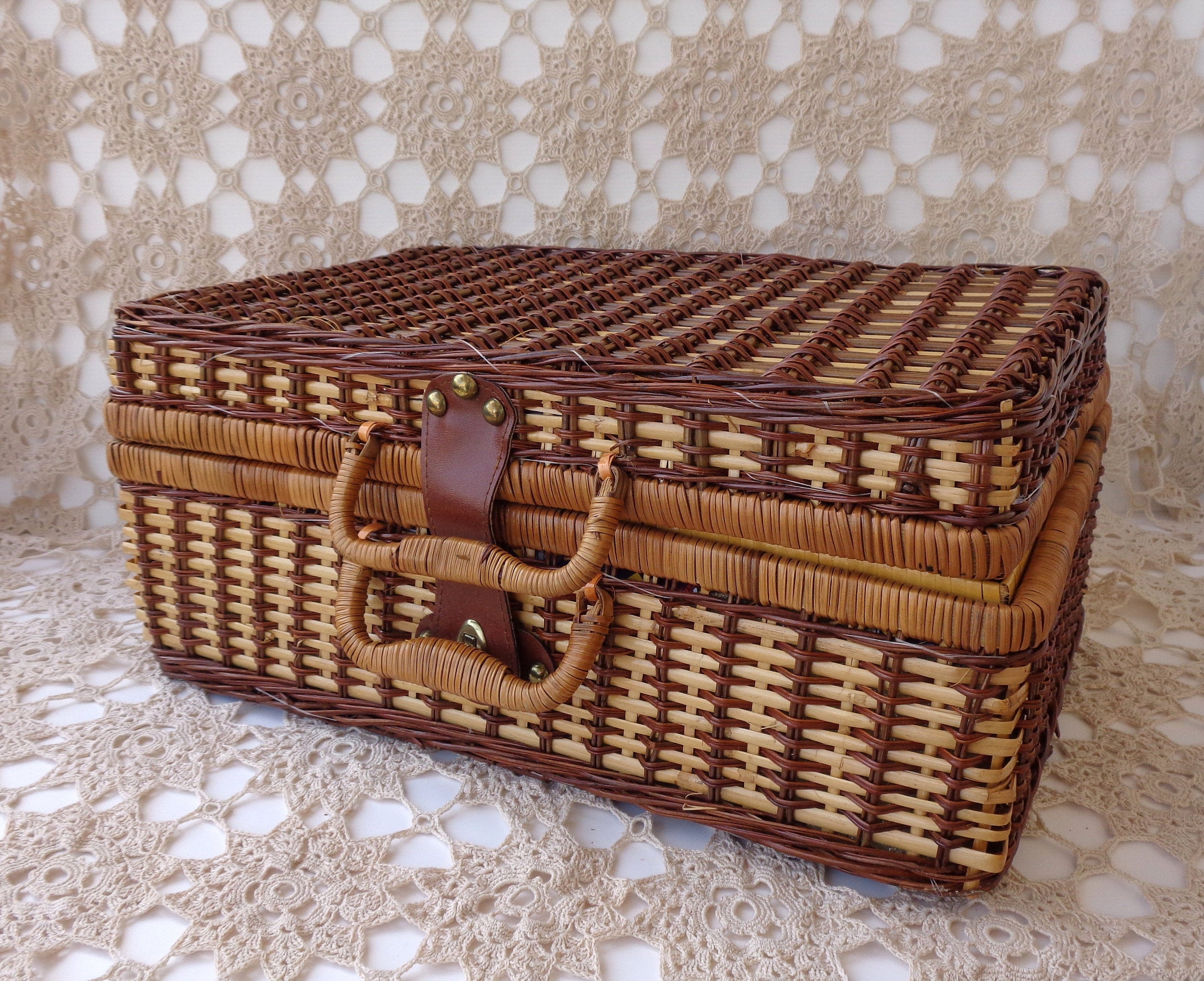This photograph features a rectangular wicker basket with a lid, crafted in a striking two-tone design. The intricate weave alternates between dark brown, medium brown, and light tan, creating a visually appealing pattern. The basket is equipped with two medium-brown handles positioned centrally, flanked by a leather strap buckle with rivets, ensuring secure closure. The basket is set atop a delicate, tan-colored, crocheted blanket adorned with a white floral pattern, while a continuation of the blanket serves as the background against a white wall. The combination of the basket's refined craftsmanship and the soft, lacy texture of the blanket adds a charming, rustic touch to the scene.